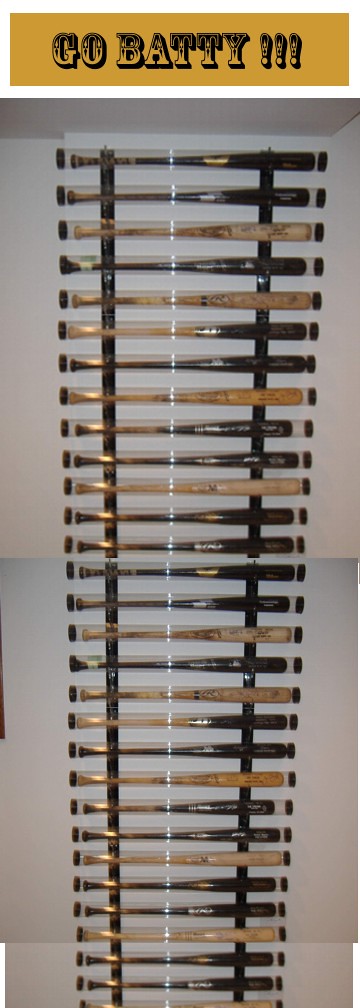The image depicts a visually striking display rack mounted on a white wall, showcasing around 40 to 50 baseball bats encased in individual translucent plastic cylinders with caps on each end. The display is horizontal, with the bats resting on hooks attached to two vertical supports. Above the rack, a digitally created banner reads "Go Batty!!!" in a black-shaded font on a gold background. The bats are arranged closely together, about one or two inches apart, and feature various shades ranging from light tan to nearly black with visible manufacturer labels. A white string runs down the front of the display, presumably to help secure the bats in place. Due to the extensive collection, the bottom edge appears to have been spliced to include all the bats in the photo.